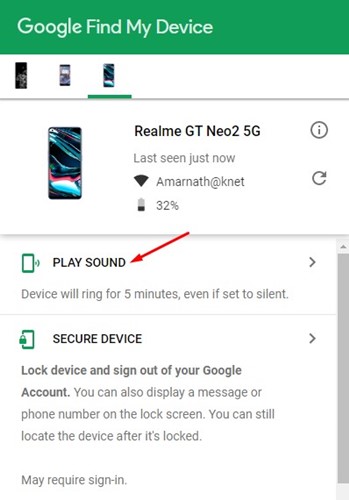The image depicts a screenshot from a mobile phone displaying the "Google Find My Device" website interface. Dominating the top portion is a green header labeled "Google Find My Device." Below this header, three devices are listed in various sizes, with the third device from the right being highlighted by a green underline.

This highlighted device appears with intricate designs featuring colors such as red, white, and blue. The device is identified as a "Realme GT Neo 2 5G," with a status indicating it was "last seen just now." Next to this, you'll find a Wi-Fi icon with the label "Amaranth at Knet," followed by a circled icon, and a battery icon showing it is 32% charged.

Beneath these details is a "Play Sound" option, represented by a phone icon. Further down is a "Secure Device" section, indicated by an arrow pointing to the right, adjacent to an icon of a phone with a lock symbol on it. Additional device security information is listed beneath this section.